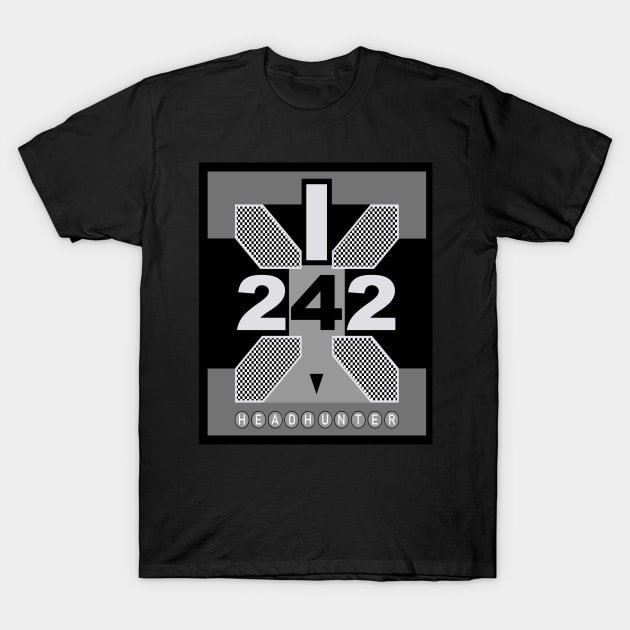This image features a black T-shirt against a white background. Centrally positioned on the T-shirt is a large square insignia with gray borders at the top and bottom. Inside the square, against a black background, are the numbers '2', '4', and '2'. The first '2' and the last '2' are white, while the '4' is black. Above each '2', there are small octagon-shaped boxes, similarly appearing below each '2'. At the top of the square, there are fin-like designs with a white stripe descending between them. Below the numbers, the fin-like designs reappear, pointing downwards toward the word "headhunter" written at the bottom of the square. The overall design gives a distinctive and detailed emblematic look to the T-shirt.